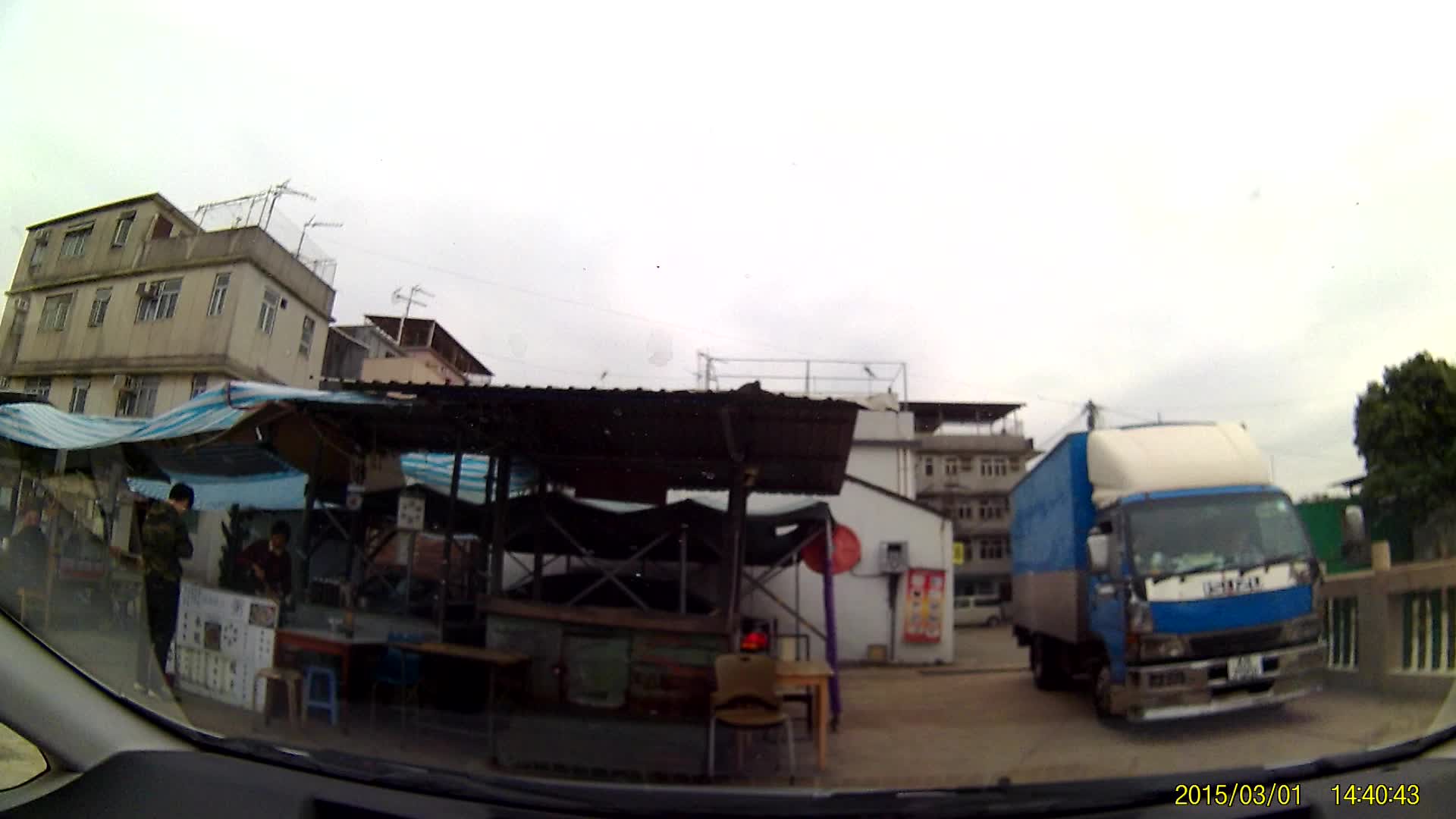This image, taken from a dash cam on March 1st, 2015, at 2:40:43 PM, captures a street scene on a cloudy day. On the left, there is a booth that appears to be an eatery where workers take their breaks. Next to it, there is what looks like a storefront with a blue tent or tarp as the roof. On the right side of the image is a large blue semi-truck. In the background, several buildings can be seen, some of which appear unfinished and unpainted. Additionally, a multi-story building with antennas on the roof is visible in the far left corner. The ground is concrete, and bits of the car’s interior dashboard are peeking into the frame, adding context to the perspective. Above, patches of the sky are visible through the clouds.